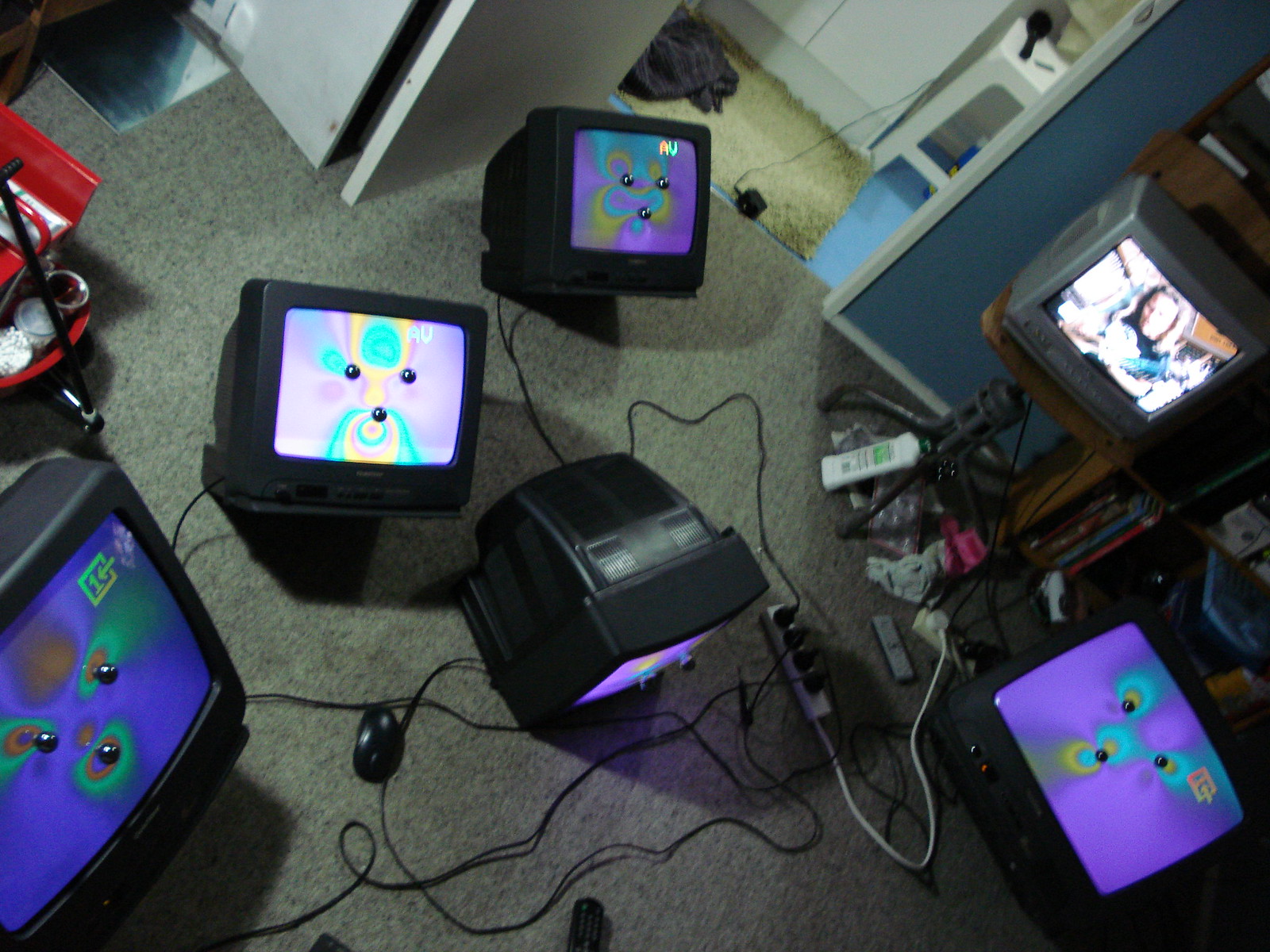The photograph captures a room with medium blue-gray painted walls and a gray carpeted floor, viewed from above. At the center of the scene are six small, black CRT tube televisions arranged haphazardly on the floor. Each TV screen displays a unique, colorful, and somewhat distorted image, with psychedelic swirls of purple, blue, and yellow hues that form simplistic faces using two dots for eyes and one dot for a nose. One of the TVs has a blurred image that's indistinguishable. The TVs are all plugged into a fully occupied surge protector, contributing to a tangle of various wires on the floor. In the background, there is a tan door, and beyond it, another room is visible with white cabinets, a yellow rug, and blue floors. The photograph, which is devoid of any text, seemingly focuses on the artistic and visual arrangement of the vintage televisions, highlighting their presence as the main subjects amidst the surrounding details.